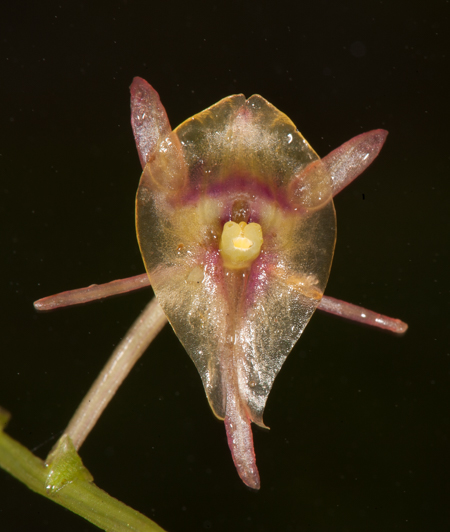This highly detailed macro photograph captures a unique and delicate plant against a completely black background peppered with faint white specks. Dominating the bottom left corner, a sturdy green stem branches out, leading to an intricate and translucent flowering structure centered in the image. The flower's petals, light pink and shiny, extend outward in a star-like formation from a central, oval-shaped bloom. This bloom, notable for its clear, golden transparency, is incredibly thin and delicate, almost membranous in appearance. A subtle purple hue and a prominent yellow centerpiece enhance its ethereal quality. The overall composition suggests a surreal, almost otherworldly plant, captured with sharp clarity and detail, highlighting the flower's unusual colors—tan, pink, purple, yellow, and green—transient shine, and delicate forms.